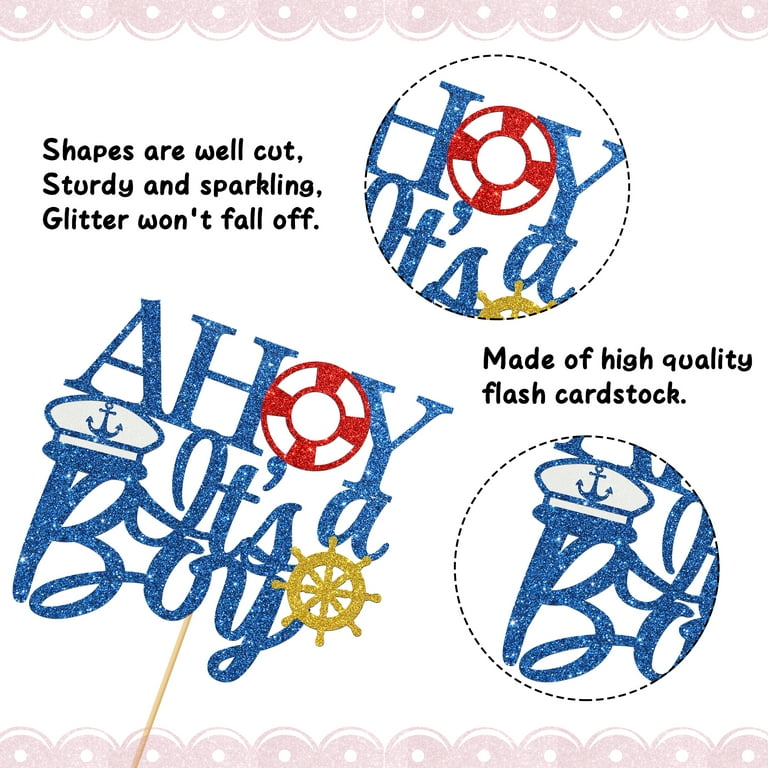The image depicts a decorative card framed by pink scalloped borders with white polka dots. The top left corner features black text stating, "Shapes are well cut, sturdy and sparkling, glitter won't fall off." Center-right, in blue glittery text, "Ahoy! It's a Boy" is prominently displayed, with creative details: a red and white life buoy for the "O" in "Ahoy," a white sailor's cap with a blue anchor embellishing the "B" in "Boy," and a golden ship wheel adjacent to the "Y." High-quality flash cardstock is used, as mentioned at the bottom left, ensuring durability and sparkle retention. Circular cutouts provide close-up views of the sailor hat and the life buoy, giving a detailed look at these charming nautical elements.